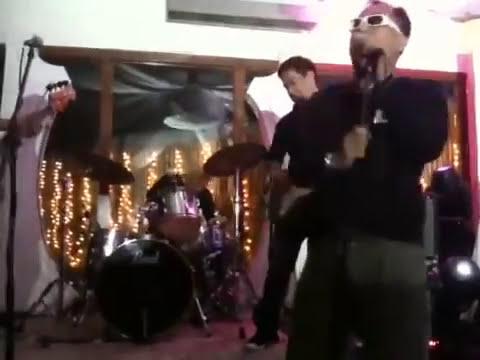The photo captures an indoor scene that is slightly blurry and appears to be of a band practice or recording session, possibly for a music video, set in what seems like a high-rise apartment with sprawling views of other skyscrapers illuminated with yellow lights visible through a large sliding glass door or window with dark brown wooden frames. In the foreground on the right side, there is an Asian man wearing white, thick-rimmed sunglasses, a black long-sleeved sweater, and dark grey pants, holding a microphone close to his face as he sings. To his left, there is another Asian man dressed entirely in black, including black shoes with white soles, who seems to be playing a guitar. Behind them, a drum set is positioned near the window. Adding to the cozy yet lively ambiance, warm golden lights, resembling Christmas lights, are strung around the staging area. The scene is set against white walls, enhancing the overall depth and sense of space in the image.